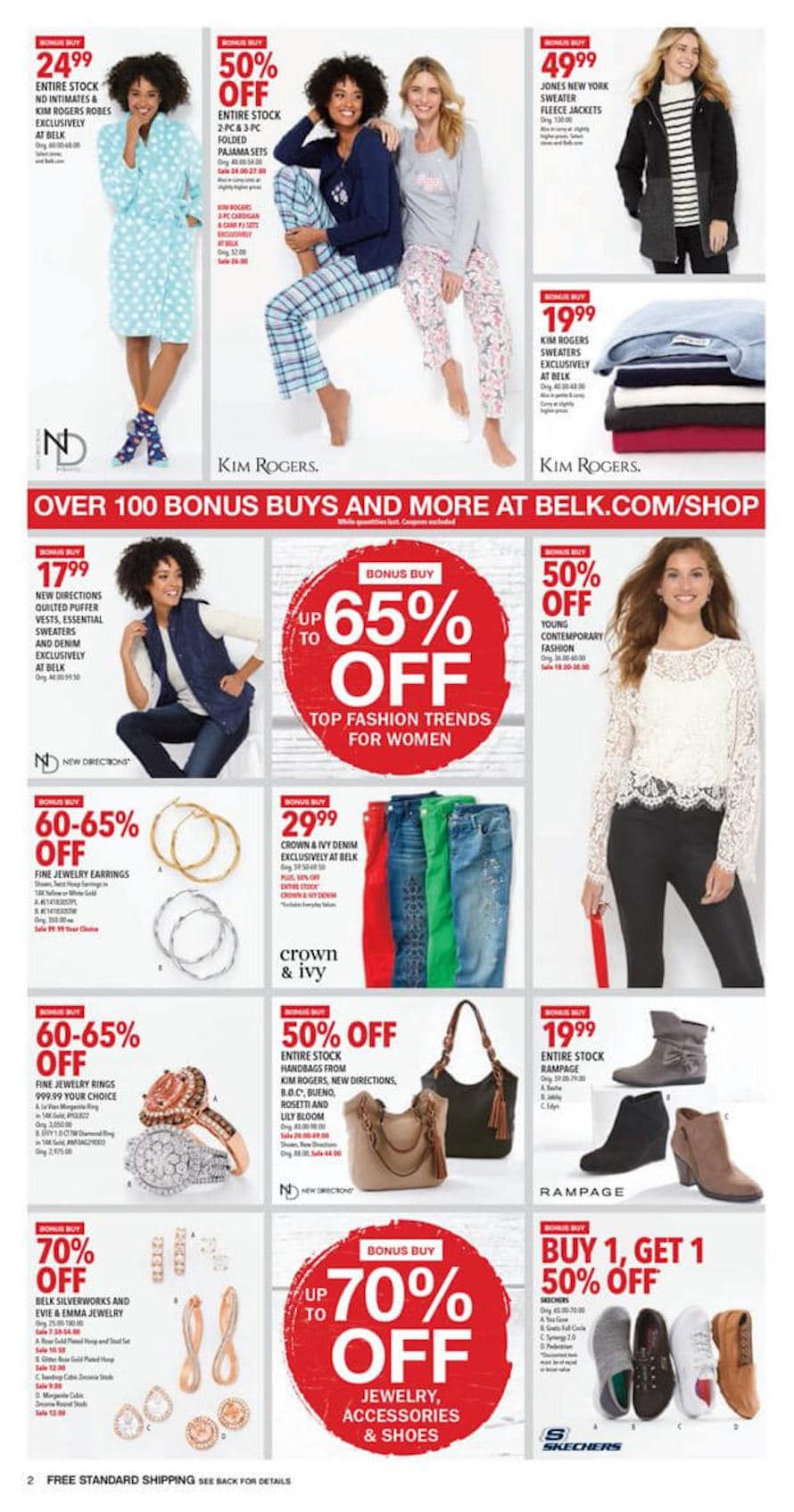The flyer, reminiscent of traditional JCPenney or Macy's advertisements found in newspapers or mailed catalogs, is now primarily available online. The bottom section of the flyer features a note in black text stating, "Free standard shipping. See back for details," accompanied by a superscript "2". 

At the top, bold red text announces "70% off jewelry" with brands like Belk Silverworks and Evie and Emma prominently featured, indicating the retailer is Belk. A central red circle with white text proclaims "Up to 70% off jewelry, accessories, and shoes."

Further down, a box highlights a "Buy one, get one 50% off" offer on TOMS and Skechers. Above this offer, "$19" is displayed in red, followed by "Entire stock Rampage" in black, showcasing various boots in gray, black, and beige. Another section announces "50% off entire stock handbags" from brands such as Ken Rogers and New Directions.

The flyer also includes a "60% off fine jewelry rings" deal, featuring items priced at $999.99. Nearby, a similar "60% off fine jewelry earrings" offer emphasizes gold and silver hoops. Denim jeans from Crown and Ivy, exclusive to Belk, are priced at $29.99 and available in red, green, and blue.

Above these sections, another red circle indicates "Up to 65% off top fashion trends for women." Lastly, the flyer promotes "50% off young contemporary fashion," including a white floral shirt.